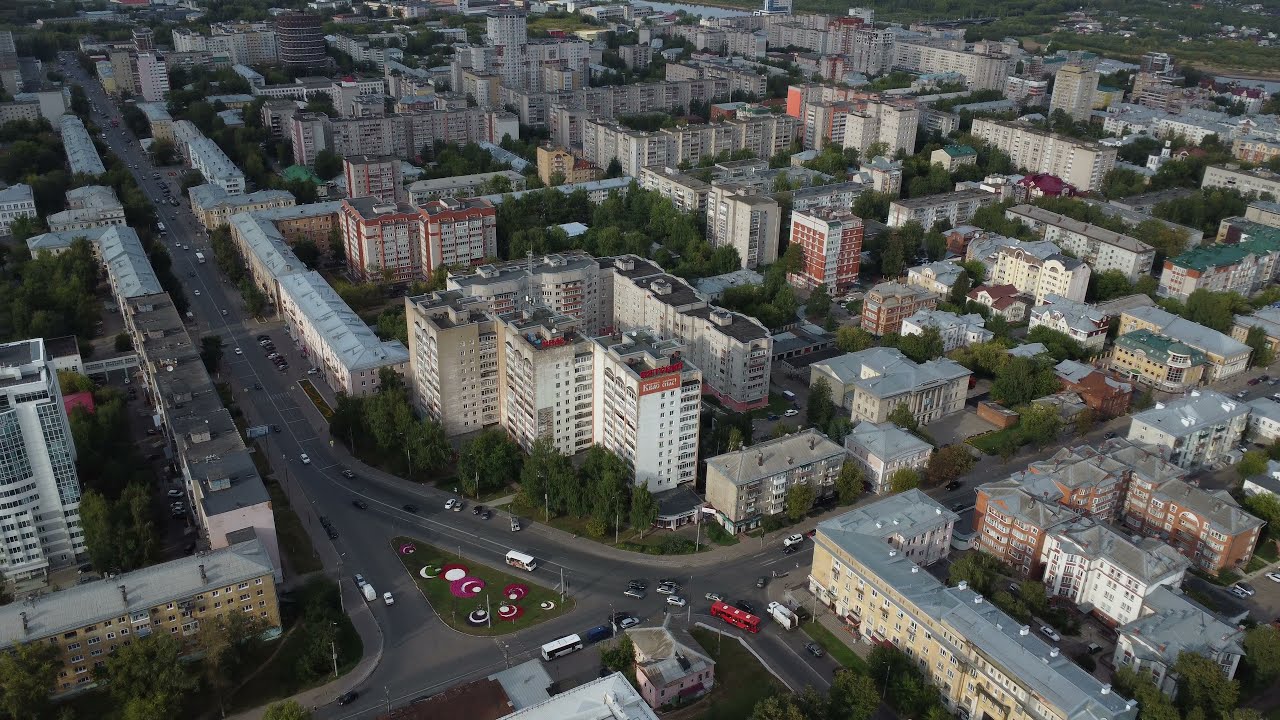This photorealistic aerial image captures a sprawling cityscape at dusk, revealing a complex urban environment. Two primary roads dominate the scene, intersecting to form a triangular patch near the bottom-left quadrant. This patch is uniquely patterned with pink, red, and white circles on a grassy area, intentionally designed as part of the roadway layout. The main road stretches from the bottom-middle to the right side, while the perpendicular road extends towards the upper left. Both roads are bustling with diverse traffic, including cars in various colors, buses, and vans.

Surrounding these roads are numerous light-colored, multi-story apartment buildings and houses, primarily in shades of white, yellow, and tan, with some featuring red and white accents. Many buildings have grayish-blue rooftops. Interspersed among the buildings, green trees provide a touch of nature within the urban sprawl. The density of buildings decreases towards the top-right, transitioning into greener, more open spaces with fewer structures. Faint natural lighting suggests the image was captured around dusk, highlighting the intricate details and colors of this vibrant city center.